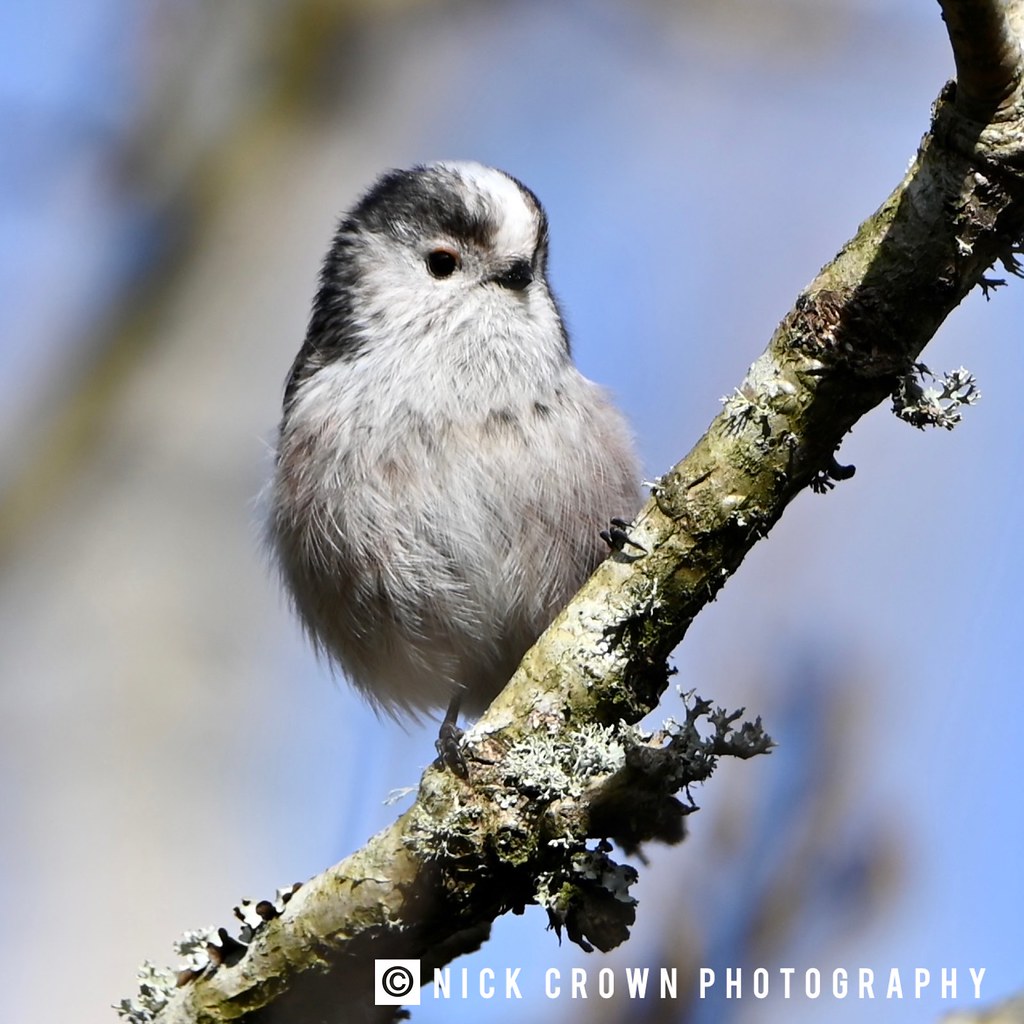The vividly detailed photograph showcases a small, plump bird perched centrally on a greenish gray branch, which diagonally spans from the bottom left corner to the top right corner of the frame. The branch is aged, with various green and white organic growths texture its surface. The bird's short, black legs firmly anchor it to the branch. Its body is predominantly whitish gray with a soft, fuzzy appearance. White spots speckle around its face and a distinct white stripe runs down the center of its head. The bird's back is a stark black, contrasting with its small, pointed black beak and tiny black eyes. The overall scene is set against a blurred, blue sky backdrop, creating a bokeh effect that emphasizes the bird's delicate features. In the bottom right corner of the image is a watermark that reads, "Copyright Nick Crown Photography."